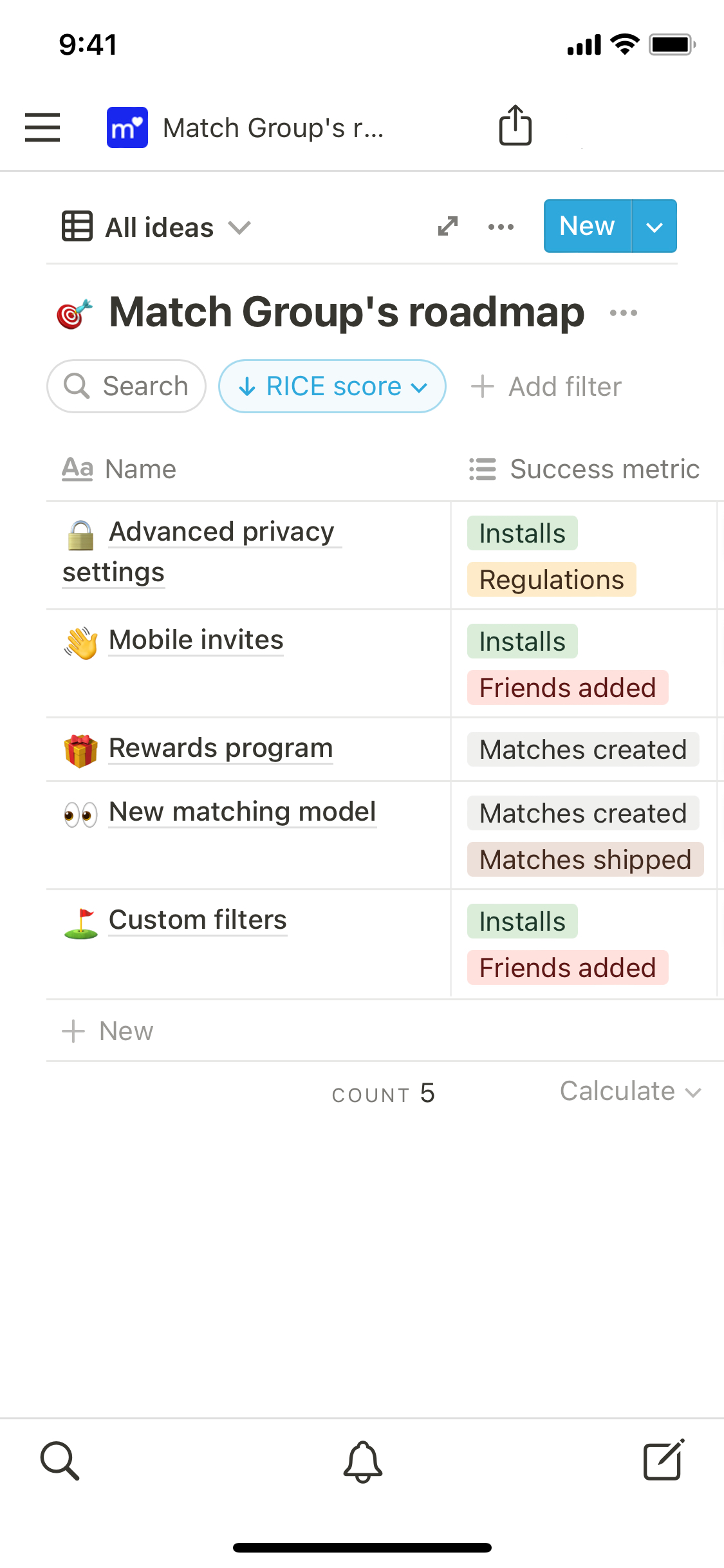This is a detailed screenshot of a cell phone display with a white background, showcasing a productivity or project management app. 

In the top left corner, the time is displayed as 9:41 a.m. The top right corner includes icons for signal strength, Wi-Fi connectivity, and battery status.

Below the status bar, on the left edge of the screen, there are three horizontal lines indicating a menu. Adjacent to this is a blue square logo with a white lowercase "m," and a caption next to it seems to read "Match Groups." Following this is a share icon represented by a square with an upward arrow inside it. 

Below this header section, a thin gray line separates it from the main content area. The first line of content features a dropdown menu labeled "All Ideas," and to its right, a "New" button with a dropdown option. Underneath this, a bullseye emoji precedes the text "Match Groups Roadmap." 

A search bar is centrally located, accompanied by a "Down Arrow" button labeled "RICE Score" and an "Add Filter" option. The main content is divided into two columns: "Name" and "Success Metric."

1. **Advanced Privacy Settings**:
   - Icon: Padlock
   - Success Metrics: 
     - Installs (green)
     - Regulations (orange)

2. **Mobile Invites**:
   - Success Metrics: 
     - Installs (green)
     - Friends Added (red)

3. **Rewards Program**:
   - Icon: Gift
   - Success Metric: Matches Created

4. **New Matching Model**:
   - Icon: Two Eyeballs
   - Success Metrics:
     - Matches Created (text on gray)
     - Matches Shipped (brownie beige)

5. **Custom Filters**:
   - Icon: Golf Course
   - Success Metrics:
     - Installs (green)
     - Friends Added (red)

At the bottom, the count is shown as "5" in the center, with a dropdown arrow labeled "Calculate" on the far right. The footer of the screenshot is marked by another thin gray line.

Below this footer line, the navigation bar features three icons: a magnifying glass for search (left), a bell for notifications (center), and an option to add a listing (right).